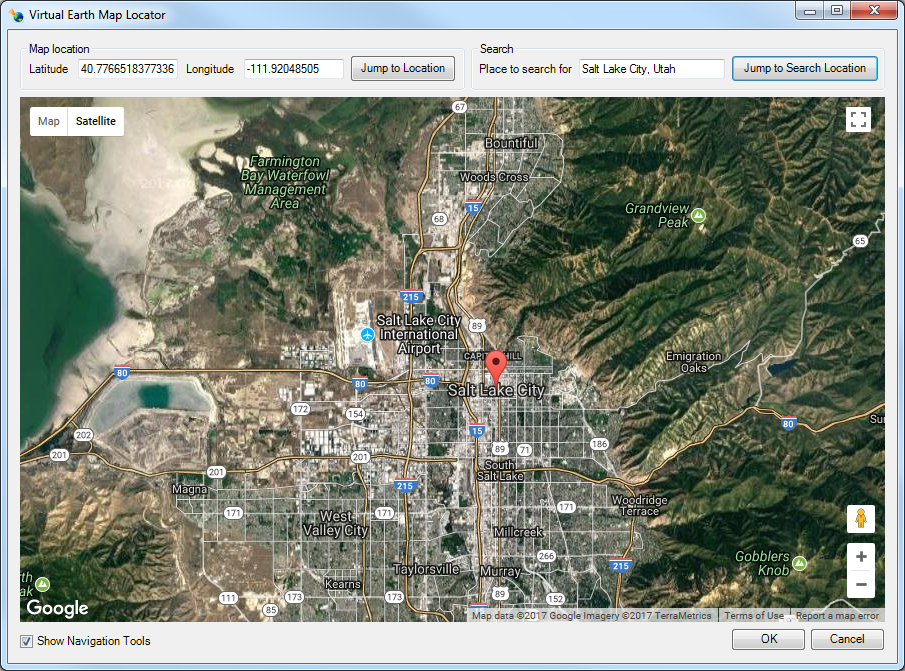**Detailed Caption:**

The image is a screenshot from a computer monitor displaying a virtual mapping tool identified as "Virtual Earth Map Locator," indicated by a blue banner at the top. The banner includes standard window control buttons: minimize, full screen, and a red close button. Below the banner, the interface shows input fields for latitude and longitude featuring long numerical strings. Adjacent to these fields is a gray box labeled "Jump to Location," accompanied by a search bar with the text "Salt Lake City, Utah." A button labeled "Jump to Search Location" is also present.

Within the map display itself, notable locations are marked: "Farmington Bay Waterfowl Management Area" is prominently displayed at the top left, with "Grandview Peak" mentioned along the bottom, and "Gobblers Knob" further down. Various city names like West Valley City, Kearns, Taylorsville, Murray, Mill Creek, South Salt Lake, Salt Lake City, and Salt Lake City International Airport are discernible. A small red icon marks the location of Salt Lake City, linking it to the search query.

The map's terrain is rendered in shades of brown, white, and green, with various roads depicted as squiggly lines. Notable landmarks and navigation options are detailed around the map. At the bottom of the image, a Google logo is visible, while the left-hand side features an option to "Click for Show Navigation Tools." To the right, there are "OK" and "Cancel" buttons.